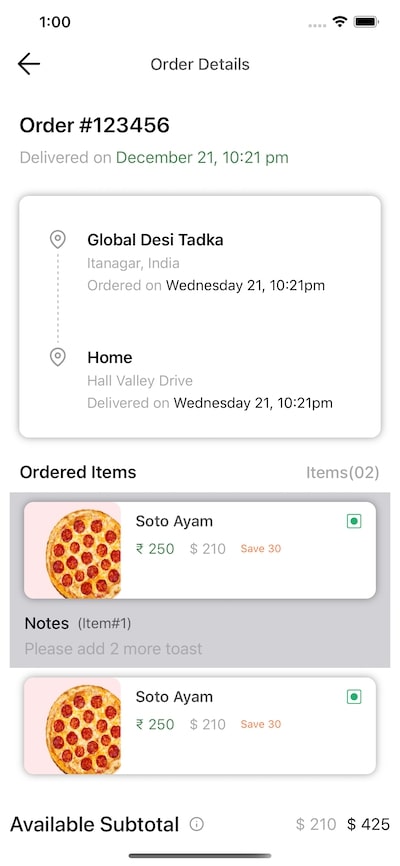**Detailed Image Caption:**

This image is a detailed screenshot of an order confirmation screen from a mobile device. At the top of the screen, the time is displayed as 1:00 (one o'clock), along with the cellular signal and Wi-Fi icons, and the battery icon indicating the device's battery level. The header reads "Order Details," with a back arrow button that allows the user to return to the previous screen.

The order is identified as Order Number 123456, which was delivered on December 21st at 10:21 PM. The order details section includes a text bar that specifies the origin and destination of the delivery: it was sent from "Global Desi TADKA" to an address on "Home Half Valley Drive," with the delivery confirmed on Wednesday, the 21st at 10:21 PM.

The itemized list of ordered goods features an icon of a pepperoni pizza, next to which the text "SOTO AYAM" is displayed, indicating one of the ordered items. There is also a promotional message in light red text, stating "Save $30." 

At the bottom of the screen, the subtotal for the available items in gray text is $210, while the total amount due in bold black text is $425, which might include additional charges or fees.